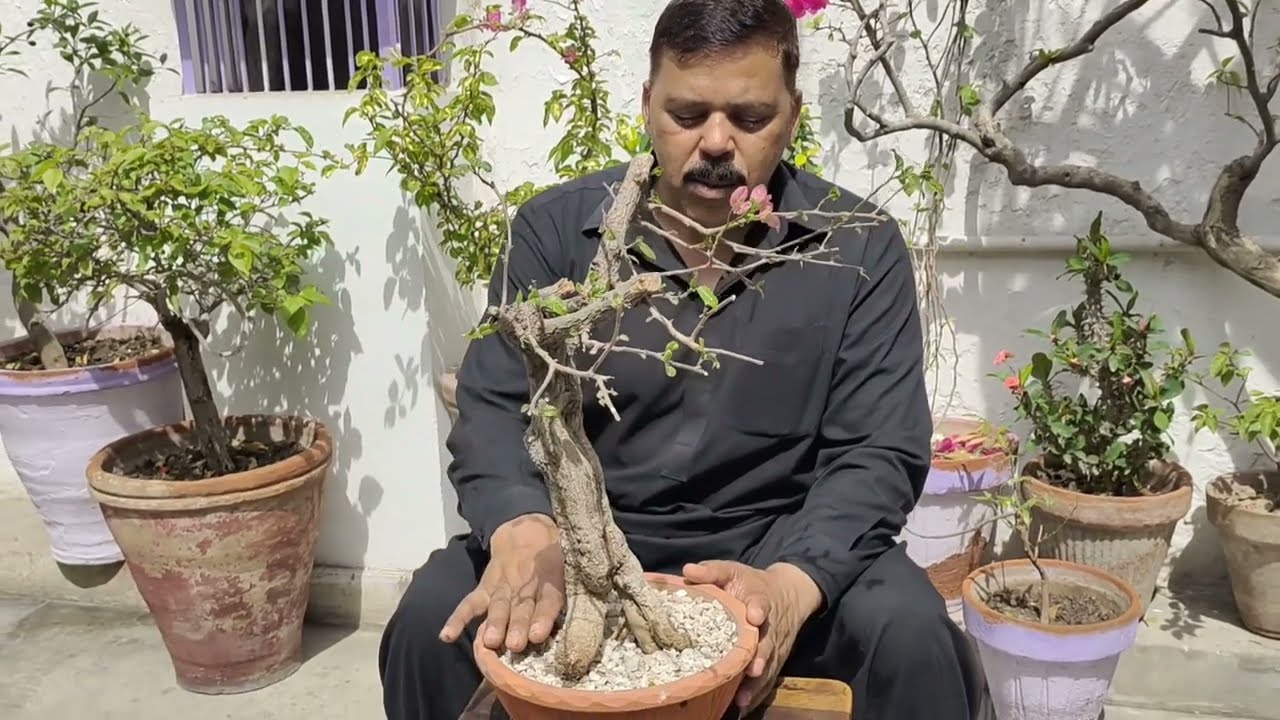The image depicts a South Asian man with a mustache and slightly balding brown hair, sitting on a bench in an outdoor garden. He is dressed in a long-sleeved gray shirt and gray pants. Centrally positioned in the image, he is holding a reddish-brown pot with a small tree that has thick, strong branches and green leaves. The pot appears to contain light soil or rocks, and the man seems to be patting down the material. Flanking him on both sides are several other potted plants. Behind him, the setting is marked by a yellowish beige building wall featuring windows with vertical iron bars. The ground is concrete, and the scene is brightened by sunlight, suggesting it is taken in the middle of the day.